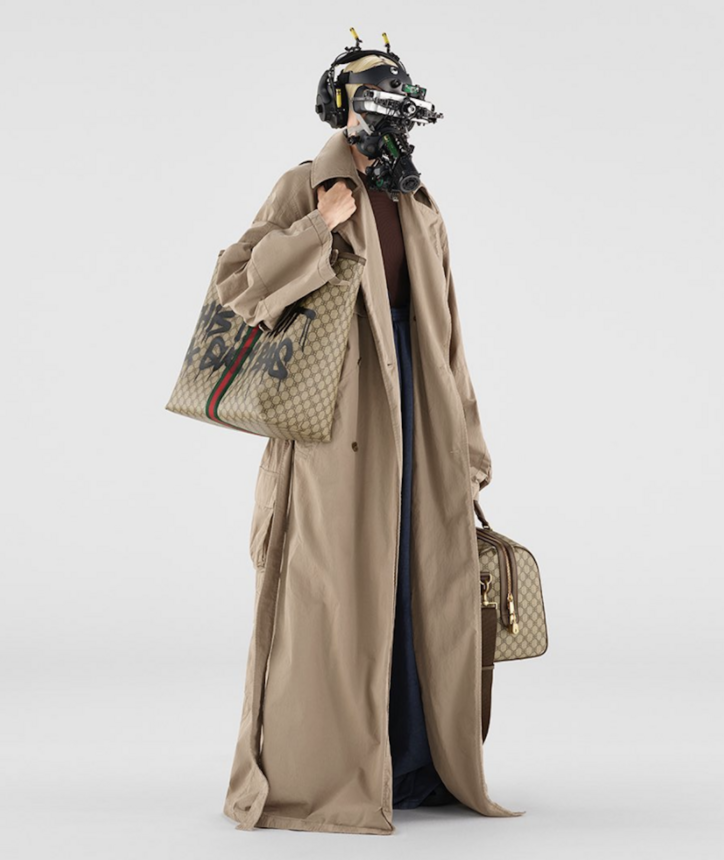The image depicts a striking cyberpunk-inspired scene with a woman standing against a seamless white background and floor, creating a stark contrast to her elaborate attire. She wears a long, light brown trench coat that reaches the ground, open to reveal a brown top paired with blue denim bottoms. Her outfit is accessorized with two notable bags: a large, tan Gucci handbag with green and red vertical stripes and black graffiti-like writing on it, slung over her right shoulder, and a matching brown travel bag in her left hand. The most arresting feature is the robotic mask covering her face, resembling a sophisticated VR headset. This device includes black headphones over her ears, a multi-colored eyepiece with hints of white, green, and yellow, and a cylindrical component at her mouth that could be a sensor or a rebreather. Her blonde hair is adorned with two yellow antennas, completing her futuristic appearance.